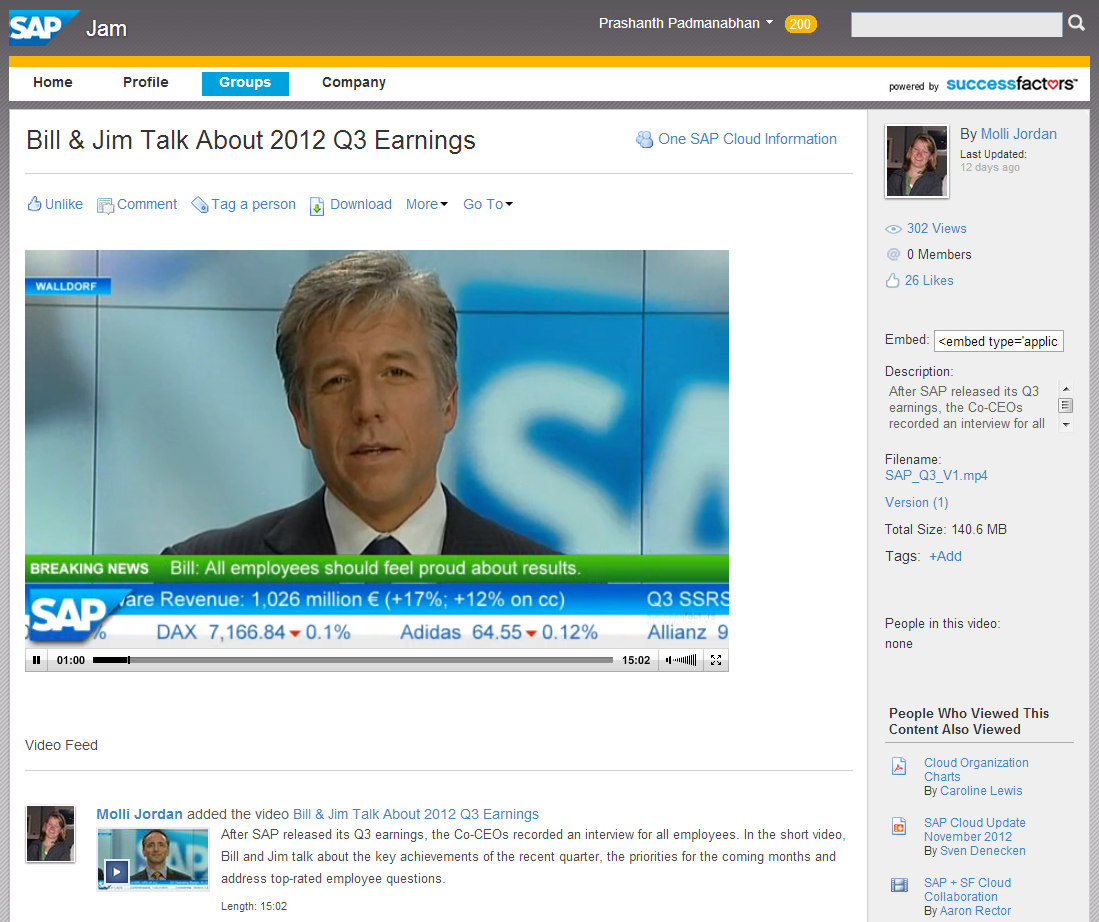**Detailed Caption:**

In this image, the top left corner displays the corporate logo "SAP" in white, set against a blue background, while immediately to its right, the word "gem" is shown on a gray background. At the top right corner, a drop-down menu lists the names: Prashant, Petman, Aban, and Sage 200. Adjacent to this menu, a search bar is positioned. Below the search bar, the phrase "Powered by Success Vectors" is noted, with "Success" in blue, "Vectors" in black, and a red heart symbol replacing the 'O'.

On the left side, a vertical navigation menu features tabs labeled "Home," "Profile," "Groups," and "Company," with the "Groups" tab highlighted in blue, while the others remain black. Directly below this navigation, there is a caption stating, "Bill and Jim talk about 2012 Q3 earnings." To its right, the text "One SAP account information" is visible. Below this, a row of blue buttons is featured, offering options such as "Unlike," "Comment," "Tag a Person," "Download," and "Go To."

Central in the image is a picture of a man dressed in a black suit and a white t-shirt. Behind him, multiple screens display the phrase "Breaking News: Bill, all employees should feel proud about the results." Below this message, statistics indicate: "SAP revenue 1.026 million euros, +17%, +12% on CC," and stock values: "DEX 7.7166.84, -0.1%," "Adidas 64.55, +0.12%."

Towards the bottom of the image, the text reads: "Video feed: More details are added in the video. Bill and Jim talk about 2012 Q3 earnings. After SAP released its Q3 earnings, the CEO's office recorded an interview for all employees in a short video. Bill and Jim talk about the key achievements of the recent quarter, the priorities for the coming month, and address top-rated employee questions. Length: 15:02."

On the right side, a side menu includes information about the file: "By Modly Jordan, the author. Last updated 12 days ago. Trailing in two views, zero members, and 26 likes." Additionally, the file name is "SAP Q3 v1.mp4," with a version number of 1, a file size of 140.6 megabytes, and a note that there are no people in this video.